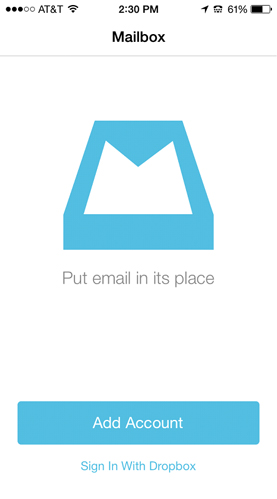The image features a primarily white background, highlighting several distinct elements. 

In the top and left sections, there are five circles aligned vertically. The first three circles on the left are entirely black, while the last two are split with a white center and a black border. Adjacent to these circles, the black text "AT" is displayed alongside a hand symbol for the letter "T." Additionally, Wi-Fi signal bars are visible, with black lines extending across them.

Central to the image, the current time is displayed in bold black text as "2:30 PM." Directly beneath this, the word "MAILBOX" (all capitalized) is prominently featured, followed by a symbol.

In the top-right corner, an arrow pointing diagonally to the right is depicted in black, though its exact purpose is ambiguous. Beside the arrow, the battery indicator shows 61% charge, with the majority of the battery icon filled in black and the remaining 39% appearing white.

Below the "MAILBOX" label, a thin gray border separates the upper and lower sections of the image. Under this border, a blue rectangle contains a white outline of two mountain peaks. Beneath this illustration, the text "Put email in its place" is displayed in black, with each word’s initial letter capitalized.

Further down, a light blue rectangle shows "Add Account" in white text, with each word beginning with a capital letter. At the bottom, another light blue section reads "Sign in with Dropbox," with the initial letters of "Sign," "in," "with," and "Dropbox" capitalized.